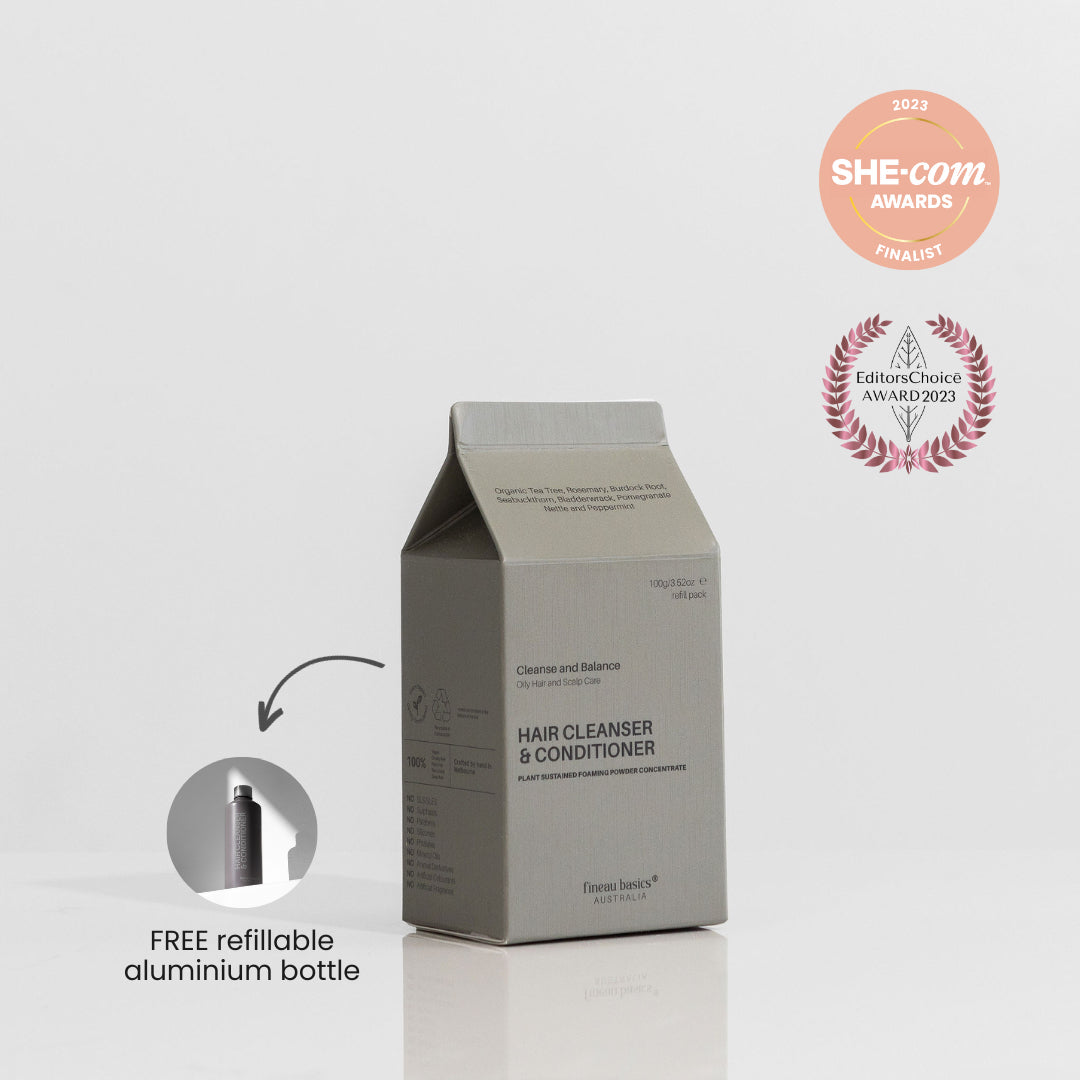The image is an advertisement for a hair cleanser and conditioner by Finu Basics, Australia. At the center is a tan-gray container resembling a small milk carton. The carton is covered in descriptive text, prominently displaying "Hair Cleanser and Conditioner" along with "Cleanse and Balance" at the top and "Plant" lower down. To the left of the carton, a gray arrow points to an illustration of a grayish-black aluminum bottle with the accompanying text "Free Refillable Aluminum Bottle." Both the product and the background are set against a white, glossy surface. In the upper right corner, there are two award insignias: a pink circle stating "2023 SHE.COM Awards Finalist" and another circle with a braided flower insignia indicating "Editor's Choice Award 2023."